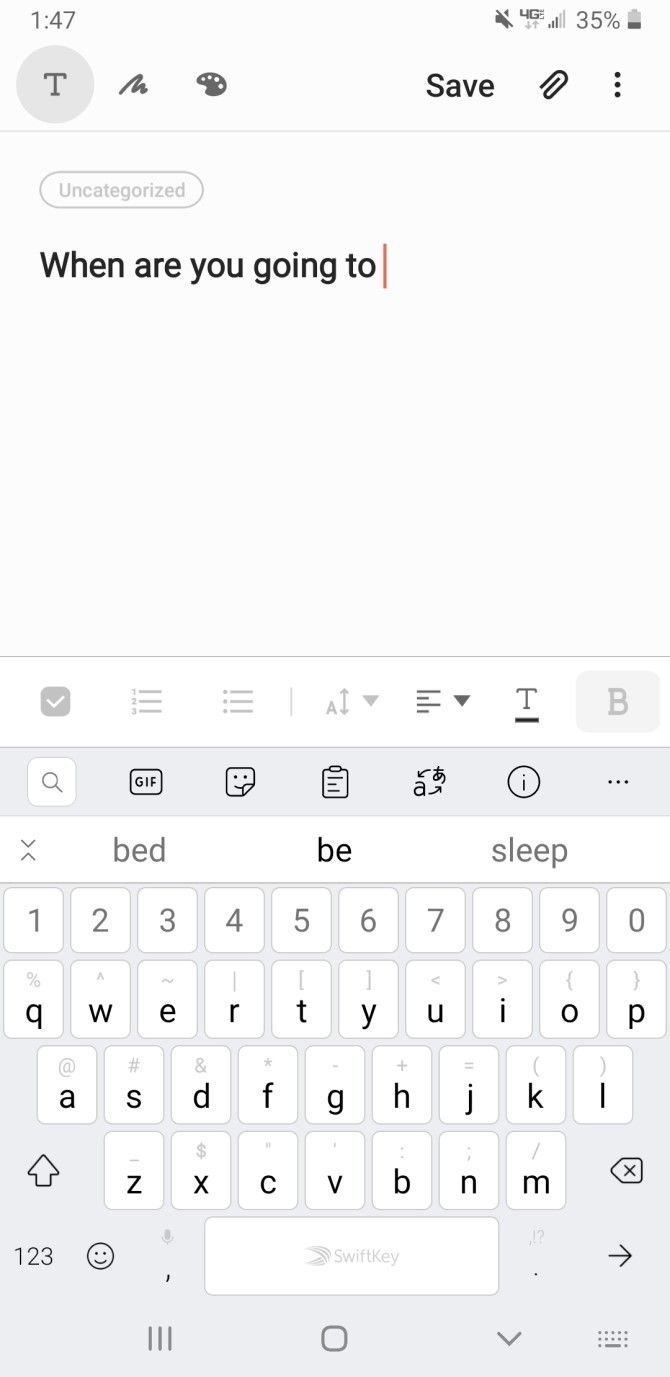This screenshot, captured from a smartphone, depicts a text message being composed. At the top, the device's status bar displays the time as 1:47 in dark gray, while the right-hand side shows various icons: a muted notification symbol, signal bars, and a battery icon indicating 35% charge, with the numerical battery level also stated as 35%. Below the status bar, the message composition area features bold black text reading "Where are you going to?" accompanied by a vertical orange line. At the bottom of the screen, a standard smartphone keyboard is present, complete with autocorrect suggestions above it. Above the suggestions, a row of icons includes options for search, GIFs, emojis, clipboard access, a formatting icon with an "A" and arrows, an information circle icon, and a menu represented by three vertical dots for additional options.